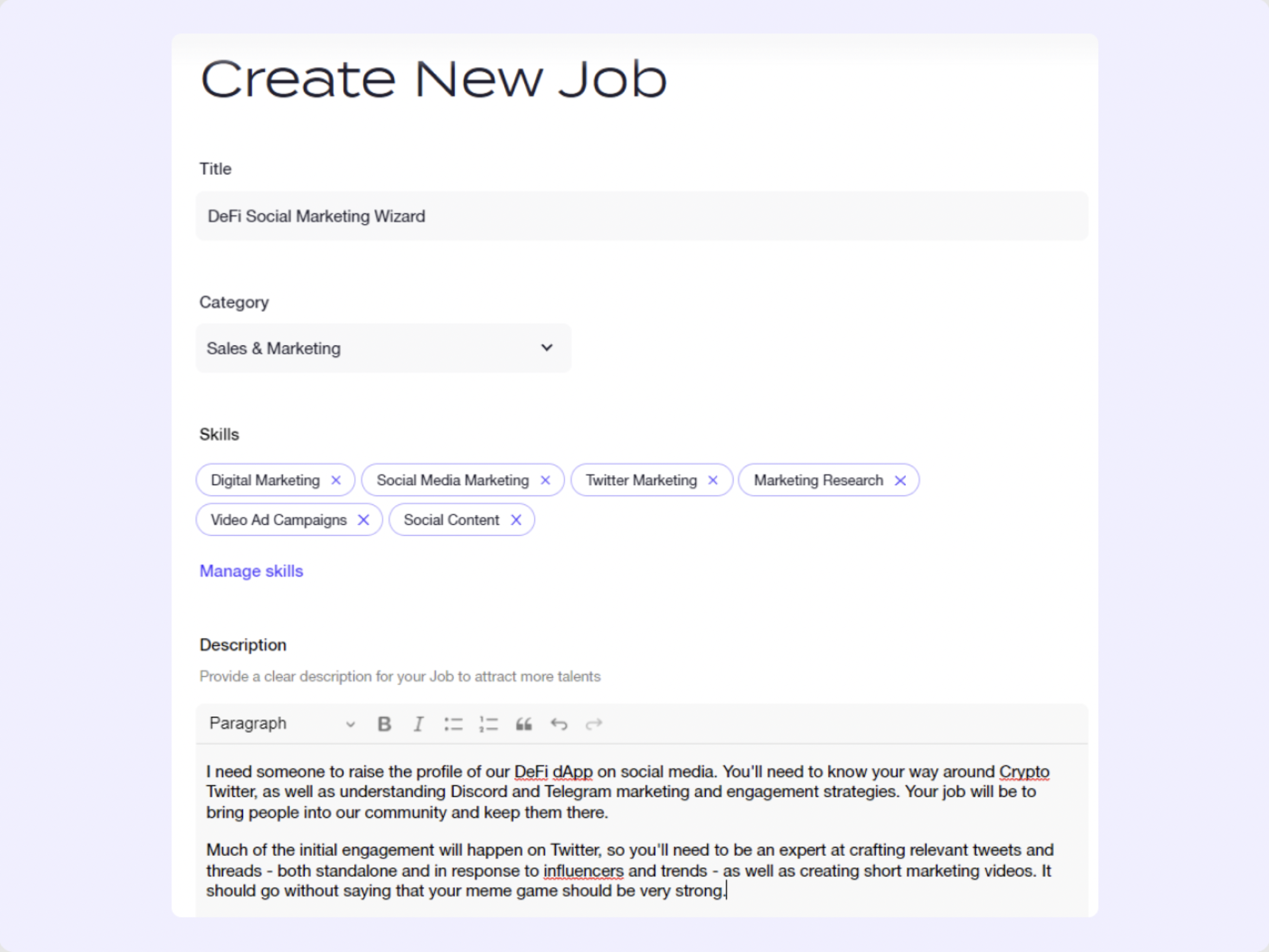The image displays an online job creation form titled "Create New Job." The job title is specified as "DeFi Social Marketing Wizard." In the category dropdown box, "Sales and Marketing" is selected. Underneath the skills section, various tags are listed, including "Digital Marketing," "Social Media Marketing," "Twitter Marketing," "Marketing Research," "Video Ad Campaigns," and "Social Content." A prominent purple button labeled "Manage Skills" is present.

The description section prompts users to "Provide a clear description for your job to attract more talents." The text box includes options to adjust settings, with formatting tools such as bold and italics, and navigational arrows for undo and redo actions. The box contains the following detailed job description: 

"I need someone to raise the profile of our DeFi DApp on social media. You'll need to know your way around Crypto Twitter, as well as understanding Discord and Telegram marketing and engagement strategies. Your job will be to bring people into our community and keep them there. Much of the initial engagement will happen on Twitter, so you'll need to be an expert at crafting relevant tweets and threads, both standalone and in response to influencers and trends, as well as creating short marketing videos. It goes without saying that your meme game should be very strong."